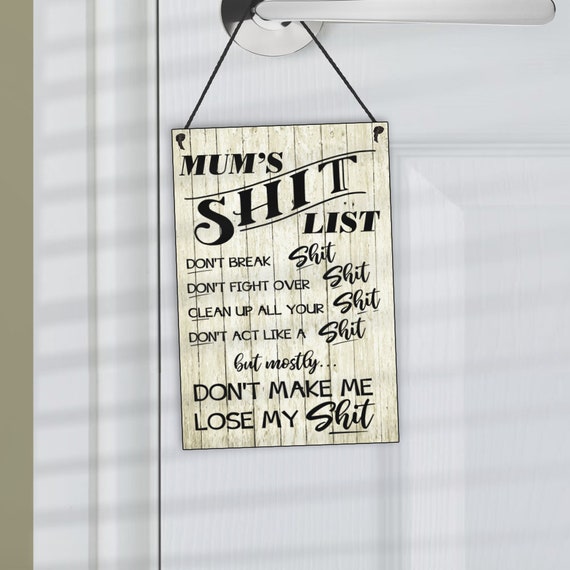The photograph captures a humorous sign titled "Mom's Shit List" hanging off a silver doorknob on a white door, framed by a white door frame. The sign, intended to look like wood, is actually made of faux wood and is beige in color. It hangs from a black string attached at the top. The list on the sign, written in black lettering, humorously outlines family rules: "Don't break shit, don't fight over shit, clean up all your shit, don't act like a shit, but mostly don't make me lose my shit," with the word "shit" underlined in each rule. The photo also shows a sliver of a beige-colored wall to the left.